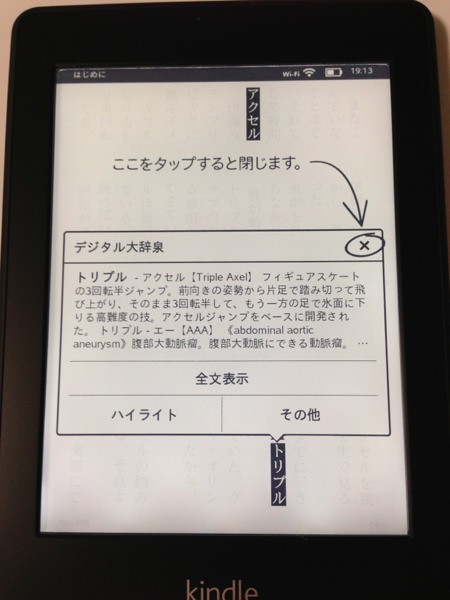The photograph depicts a black-framed Kindle device, prominently displaying the word "Kindle" at the bottom of the frame. The device is set on a tan-colored surface. The screen showcases a document written in Japanese, with notable features such as an arrow pointing downwards to an X encircled in black on a white background. Additionally, the Kindle's status bar at the top of the image indicates a Wi-Fi connection with full signal strength, a battery level around halfway, and the time stamped at 19:13. Among the Japanese text, there are intermittent English phrases, including "triple axel" and "abdominal aortic aneurysm." This suggests that the document may belong to a medical context. The overall scene hints at instructional content, possibly guiding the reader to dismiss a pop-up by clicking the X symbol.